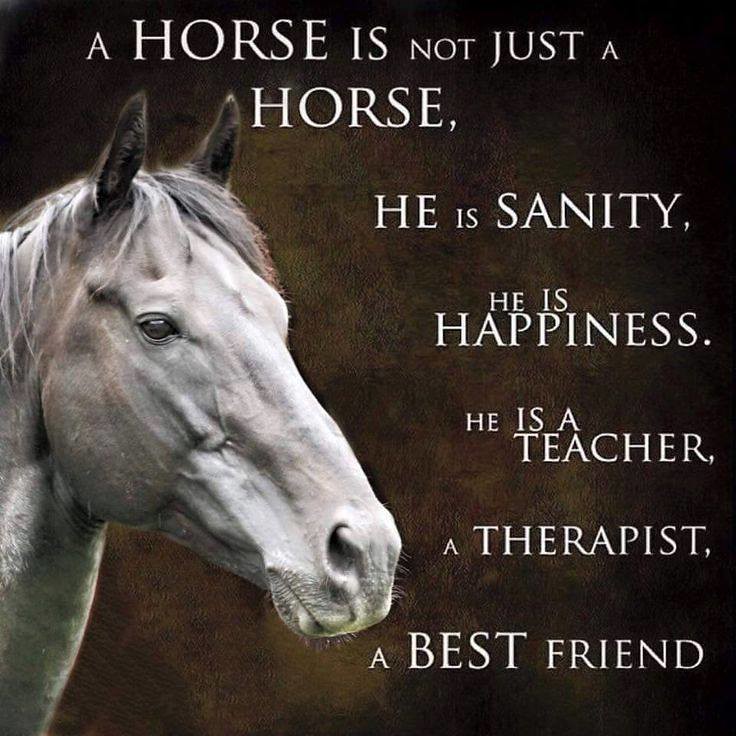This square image features a black-and-white photograph of a white horse in profile on the left side. The horse's head, characterized by long hair, is shown from the neck to the tip of its nose, with one eye visible and ears that are brown or dark-colored, creating a striking contrast. The background simulates a leather texture with a brown hue, providing a warm contrast against the monochrome subject. 

White text overlays the image, creating an impactful set of typographic statements that follow the contour of the horse's head. The text reads: "A horse is not just a horse, he is sanity, he is happiness. He is a teacher, a therapist, a best friend." This combination of photography and typography blends to deliver an inspirational and heartfelt message about the multifaceted nature of horses, highlighting their role as companions, sources of joy, teachers, and healers.